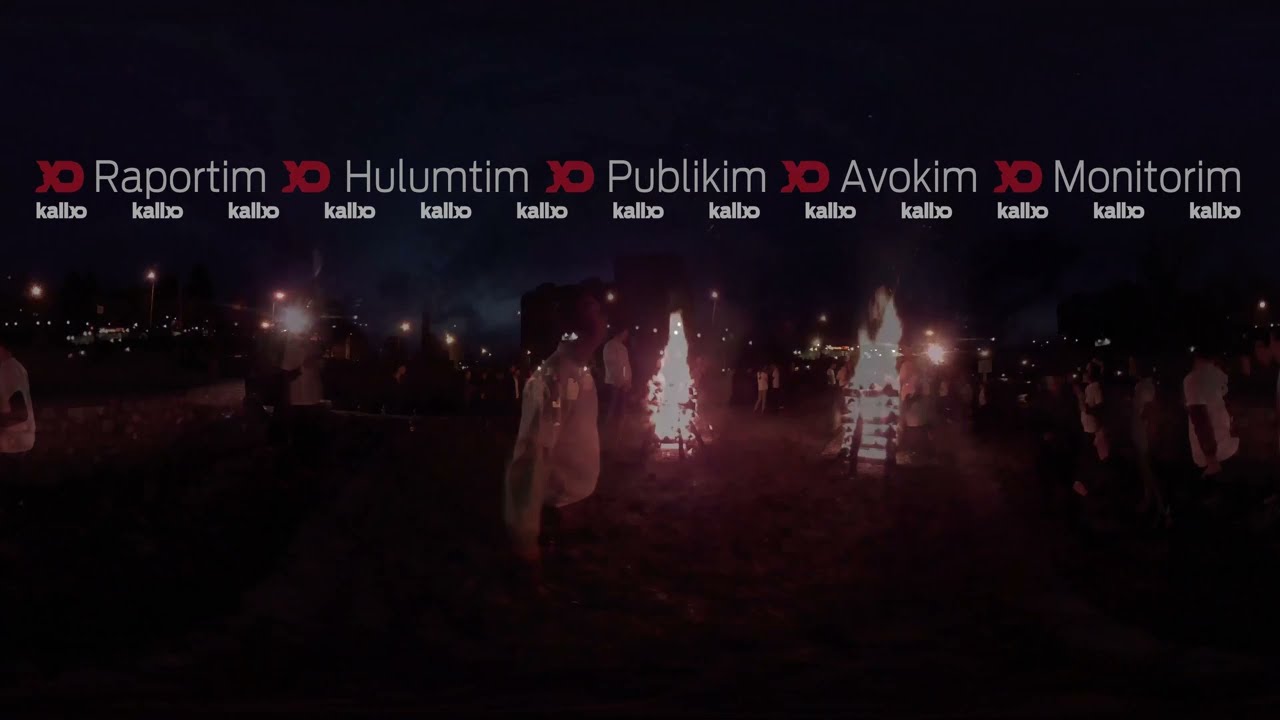In a nighttime outdoor setting, this evocative image captures a scene dominated by two central bonfires surrounded by a crowd of people. The dark sky is illuminated by the red and yellow hues of the flames, with black shadows emphasizing the night. Toward the left of the image stands a person in a white shirt, closer and more visible, adding a mysterious, almost ghostly presence due to the semi-transparent effect applied over his figure. Off in the distance, faint light poles and an empty parking lot with scattered cars are discernible on the left, while the right side showcases more people observing the fire.

Overlaying the image is a prominent banner-like text that reads "Exo Rapportim Hulutim Publicim Avokim Monitim" with a repeating "Exo" logo in red. Below this, the word "Kallo Exo" is repeated multiple times, creating a layered textual effect. The overall scene possesses an eerie yet captivating atmosphere, suggesting perhaps a ritual or significant gathering. The combination of the natural firelight, the ghostly figure, and the enigmatic foreign text enhances the surreal quality of this photograph.